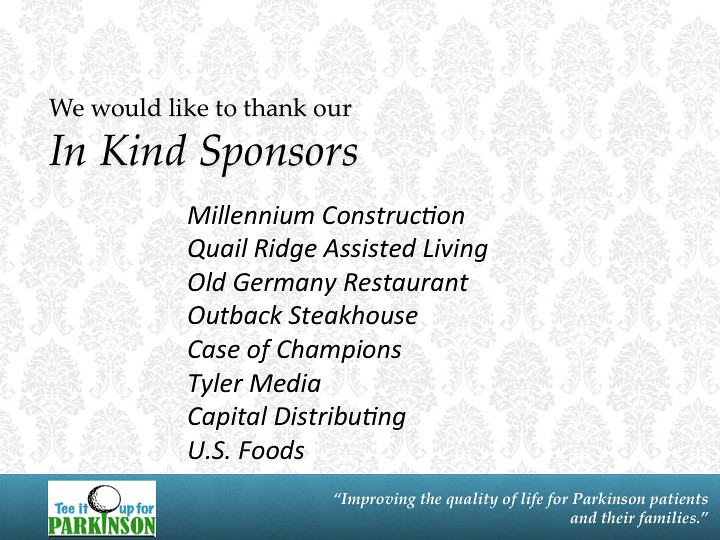This color announcement features a mostly white background with a subtle gray pattern that resembles interspersed trees. At the top of the image, a message in black ink reads, "We would like to thank our in-kind sponsors." Below this message is a list of sponsors: Millennium Construction, Quail Ridge Assisted Living, Old Germany Restaurant, Outback Steakhouse, Case of Champions, Tyler Media, Capital Distributing, and U.S. Foods. 

A medium blue banner stretches across the bottom of the image. Within this banner is a creative graphic of a golf ball perched on the letter "i" in the phrase "tee it up for Parkinson's," emphasizing the theme of a golf tournament fundraiser. The text "tee it up" is blue, while the word "Parkinson's" is green, playing on the image of a golf tee. To the far right of the banner, in quotes, the tagline reads, "Improving the quality of life for Parkinson's patients and their families." This detailed thank you note highlights the gratitude towards the sponsors for their contributions and subtly indicates the event's purpose of raising funds for Parkinson's disease.